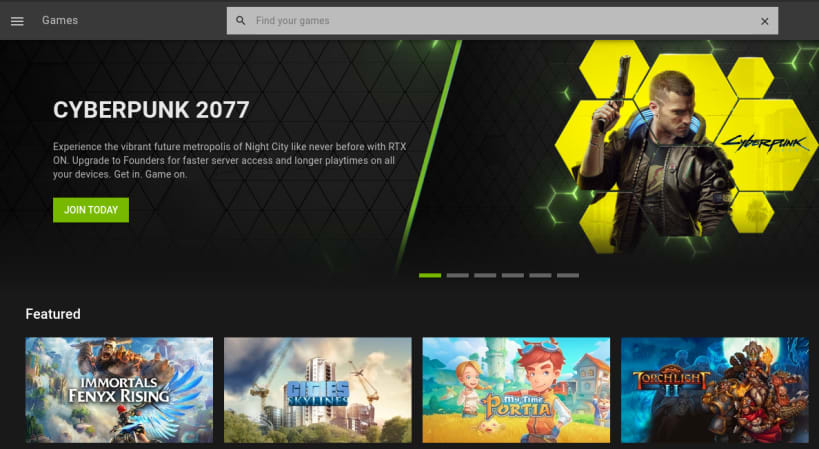The image showcases a website dedicated to "Cyberpunk 2077." The main screen features a sleek and predominantly black design with a distinct slash divider in the middle. On the left side of the slash, the text "Cyberpunk 2077" is prominently displayed at the top. Beneath it, a detailed description reads, "Experience a vibrant future metropolis of Night City like never before. With RTX on, upgrade to founders for faster server access and longer play times on all your devices. Get in-game on." Below this text, there is a striking green button that invites users to "Join Today."

On the right side of the slash, the image features a dynamic drawing of a game character. The character is holding a gun pointed straight up in the air, while his gaze is directed down at the ground to his side. The background behind the character is adorned with yellow hexagons, adding a futuristic flair to the illustration.

At the bottom of the screen, the section labeled "Featured" showcases four games. From left to right, the featured games are "Immortals Fenyx Rising," "City Skylines," "My Time at Portia," and "Torchlight II."